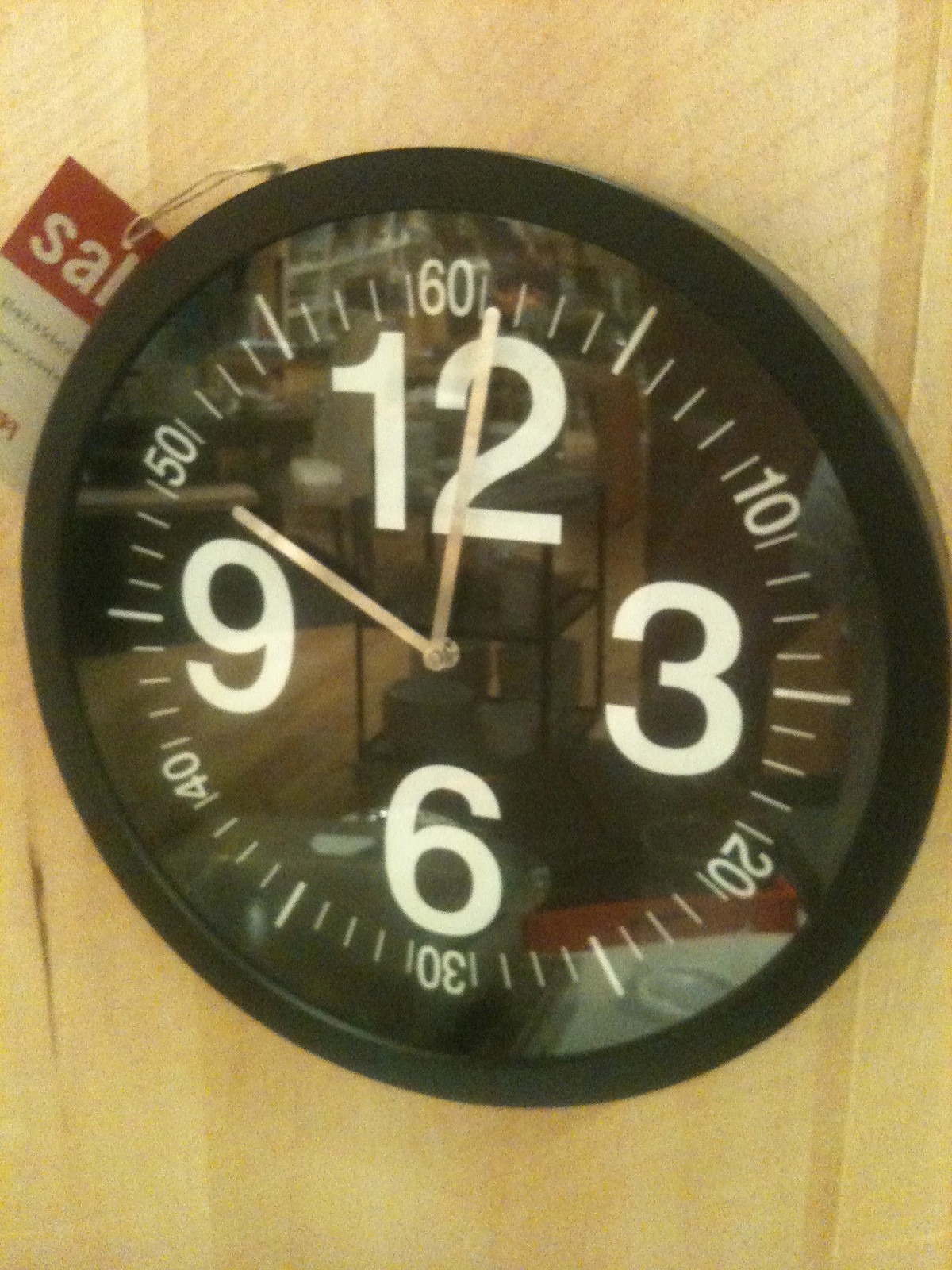A photograph capturing a black clock mounted on a wall, prominently featuring Arabic numerals. The clock is covered with a glass face that subtly reflects the room's surroundings. Attached to the clock is a red price tag, partially visible, with "SALE" written in bold white letters—only the letters "S-A-L" are clearly readable. In the reflection, various elements of the store can be seen, including shelves laden with hat boxes or round containers and additional pieces of furniture. The room's floor is made of polished hardwood, indicating the setting is a well-kept furniture store.